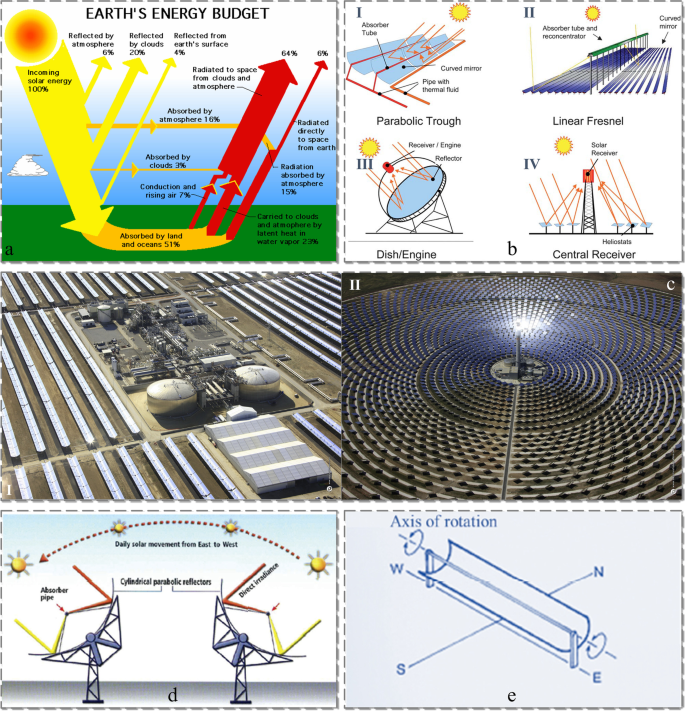The six-panel display appears to be an educational resource on solar energy systems. The top left panel, labeled A, illustrates Earth's energy budget, detailing how incoming solar energy is distributed: 51% is absorbed by land and oceans, while various percentages are reflected or absorbed by the atmosphere and clouds, with some energy radiating back into space. Adjacent to it, the top right panel, labeled B, features four diagrams of solar energy collection systems: parabolic trough, linear Fresnel, dish engine, and central receiver. These diagrams explain how curved mirrors and absorber tubes work to concentrate and absorb sunlight, with some photos providing real-life representations of these systems. The two center photos show overhead views, likely from drones, of solar farms utilizing these technologies. The bottom left panel, labeled D, depicts the daily solar movement from east to west, showing how cylindrical parabolic reflectors capture and direct sunlight throughout the day. The final panel, labeled E, illustrates the axis of rotation for these solar devices, providing a comprehensive look at their orientation relative to cardinal directions.